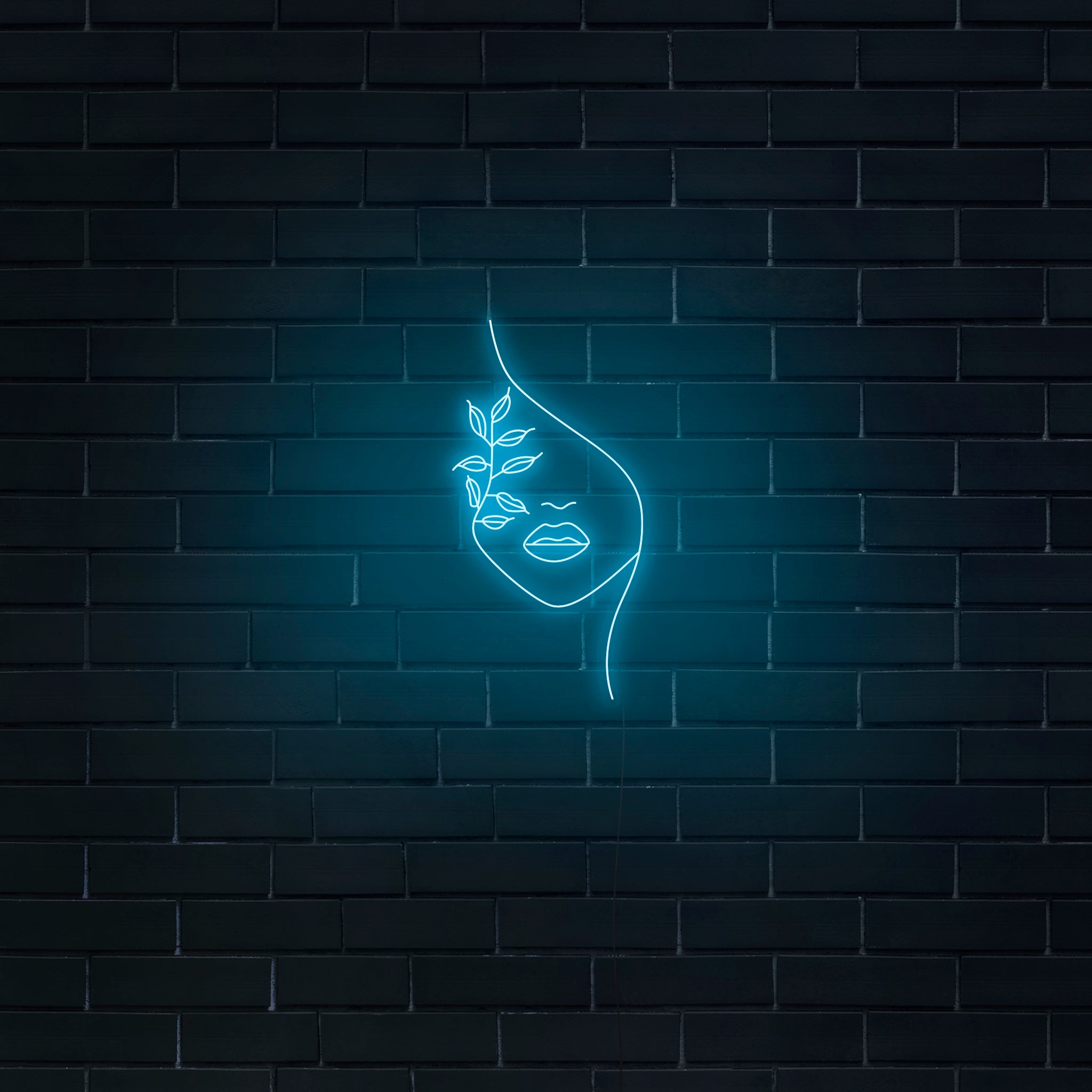The image features a vivid neon blue light display against a blue-painted brick wall, creating a striking visual effect. The illuminated graphic on the wall depicts a stylized partial face of a woman. The face is rendered with simple yet bold lines: a prominent curve for the nose, fuller lips as the main facial feature, and an outline suggesting her chin. A curving line represents her hairline. On the left side of the face, a line extends and transforms into a branch adorned with eight leaves instead of a cheek, adding a whimsical touch. The neon light enhances the blueness of the brick wall, especially where the light is most concentrated, creating an intriguing contrast with darker corners. The design extends upwards from the neck, merging the natural elements with the human face to craft an eye-catching and surreal artistic display.